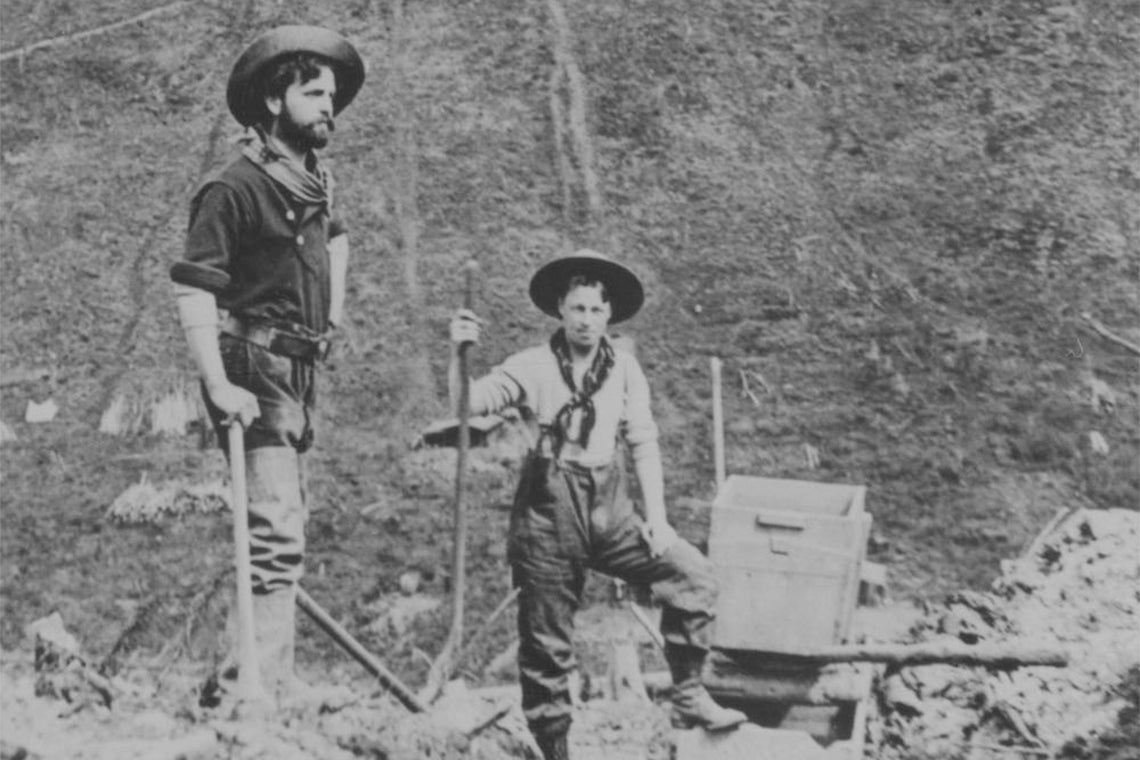This black-and-white photograph, likely from the early 1900s, captures two men standing in a barren, rocky area, seemingly in the midst of a manual labor project such as digging for a mine or well. The man on the left appears to be in his late 20s or early 30s, wearing a wide-brimmed hat tipped to the side, a beard, a dark shirt with sleeves rolled up, and lighter pants. He leans on an axe, shovel, or possibly an old fence post. The second man, positioned slightly downhill to his right, dons a similar wide-brimmed hat, a white shirt with a neckerchief tied around his neck, and darker pants. Both men lean on tools indicative of their labor, likely shovels or sticks. In the scene, there's a notable white box resting on a wooden structure and a visible hole in the ground, suggesting an active dig site. The image, devoid of plant life and filled with dirt, rock, and dust, evokes a timeless, hardworking atmosphere under bright sunlight, further emphasized by their dusty, work-worn attire suited for the harsh environment.